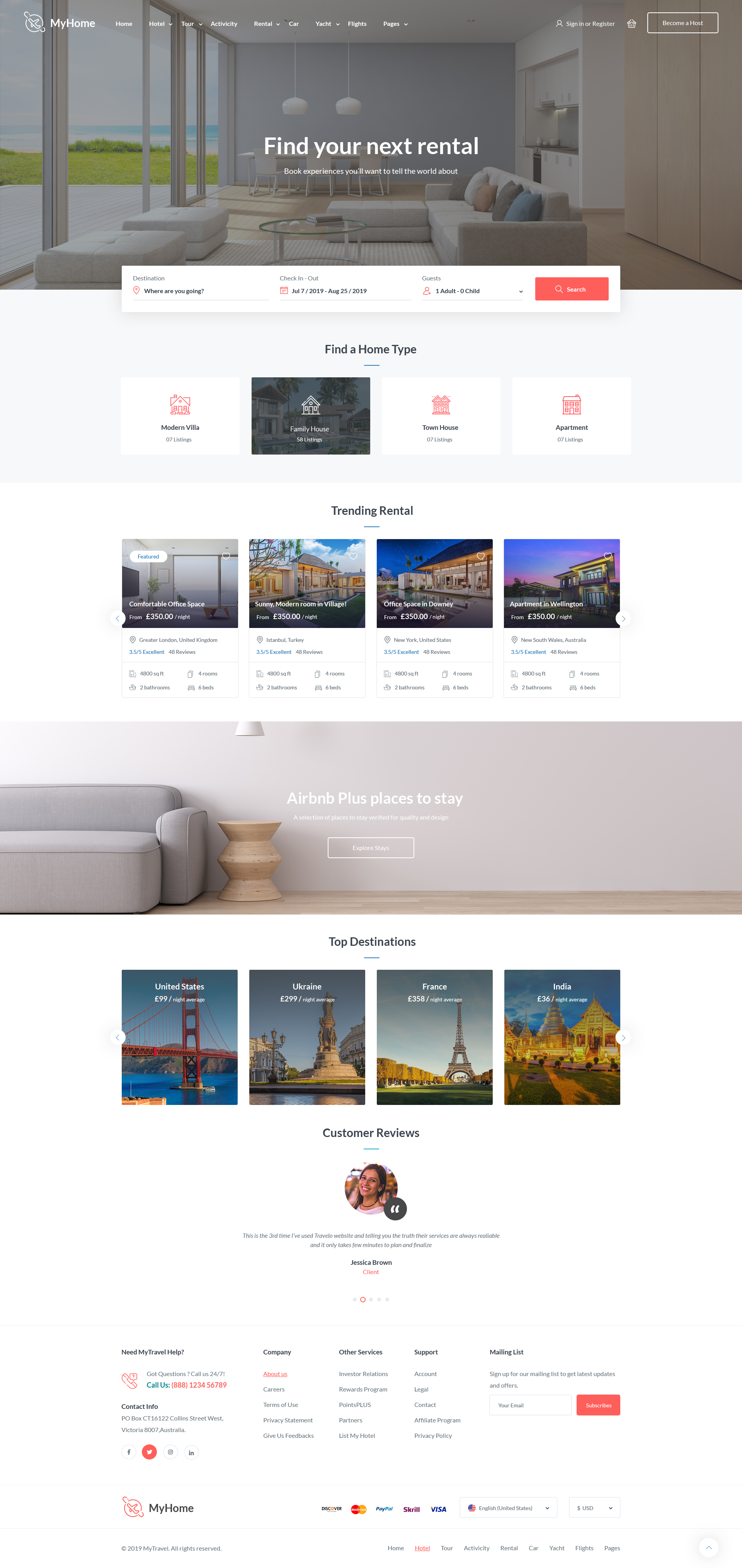The image showcases a website named "My Home," designed for renting vacation homes. At the top, there is a navigation bar featuring the website's name "My Home" along with multiple options. The header image presents a cozy living room setup. Directly beneath the navigation bar is a prominent headline, "Find Your Next Rental," followed by a short, encouraging sentence written in white letters.

The main search functionality is prominently displayed with input boxes where users can specify their destination, date range, and preferences. Below this search section lies another titled area, "Find a Home Type," featuring four distinct boxes with buttons that allow users to filter different types of homes.

Further down, the section "Trending Rentals" showcases various rental homes from cities worldwide, each accompanied by vibrant images. Following this is an image of a comfortable couch under a heading that reads, "Airbnb Plus Places to Stay," along with a white call-to-action button.

At the bottom of the page, there is a section titled "Top Destinations Around the World," listing popular travel destinations, including the United States, Ukraine, France, and India.